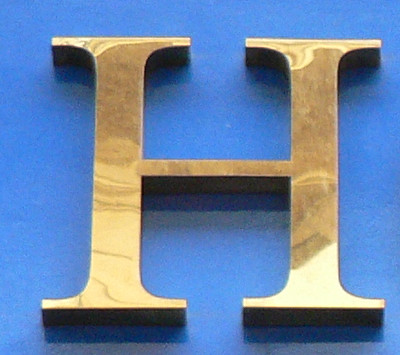This close-up photograph captures a three-dimensional, sculpted gold letter "H" mounted on a light blue wall. The "H," resembling the iconic logo of the History Channel, features intricate reflections from its surroundings, adding depth to its polished surface. Shadows cast by the "H" suggest an older image quality, possibly taken on film, evoking a sense of vintage charm. The composition is straightforward, devoid of any text or human presence, allowing the detailed craftsmanship and reflective properties of the letter "H" to dominate the visual narrative.